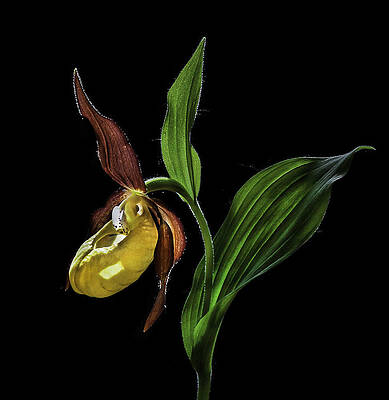The image depicts a painting of a plant, set against a pure, solid black background. The plant features a thick, green stalk that extends vertically before curving over to the left. At the bottom of the stalk, a large, green leaf extends outward to the right, showcasing detailed veining. Another elongated green leaf emerges from the top. Near the tip of the curved stalk, three narrow, reddish-brown leaves are arranged in a triangular or tripod formation. At the center of these brown leaves is a vibrant, glossy yellow bud that is bean-shaped and appears to be closed. This yellow bud, almost insect-like in appearance, shows some white highlights and reflections that suggest an artificial light source illuminating the scene from the side. The entire plant is the focus of the composition, standing out starkly against the black background, and the leaves exhibit subtle patterns and textures, adding depth and realism to the artwork.